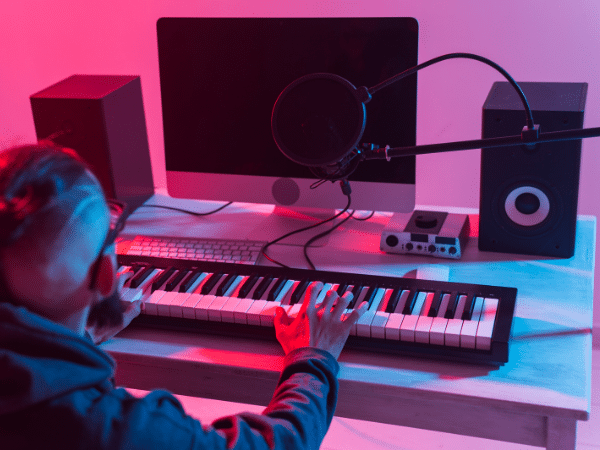In an indoor setting illuminated by a blend of striking purple and blue lights, this photograph captures a detailed scene centered around a large rectangular desk. The ambient lighting casts dramatic hues across the space, with a bright pink wall on the left and a purple one on the right. The desk, seemingly light-colored initially, morphs into shades of pink, purple, and blue due to the lighting effects.

At the heart of the image, a man, identifiable from features such as shaved sides, longer hair on top, eyeglasses, and a long beard, is seated on the left side of the desk, playing a digital musical keyboard. His hoodie, a darkish blue, contrasts with the vividly lit environment. The music keyboard keys, normally black and white, display an array of red and blue shades from the lighting.

In the center of the desk, a black monitor with a white base commands attention, flanked by two rectangular black speakers. On the right side, a grey amplifier machine with black dials is partially visible. Additionally, a small black boom mic stand protrudes from the right side towards the man. A small QWERTY keyboard is positioned near the left speaker.

The interplay of colored lights not only affects the overall atmosphere but also alters the appearance of objects and the man's hands, giving parts of his fingertips an unusual red, blue, and orange tint. This creates a surreal, almost 3D effect, making the scene feel both vividly real and slightly distorted. The meticulous arrangement and the distinct elements make this photograph a compelling snapshot of a highly personalized and illuminated workspace.